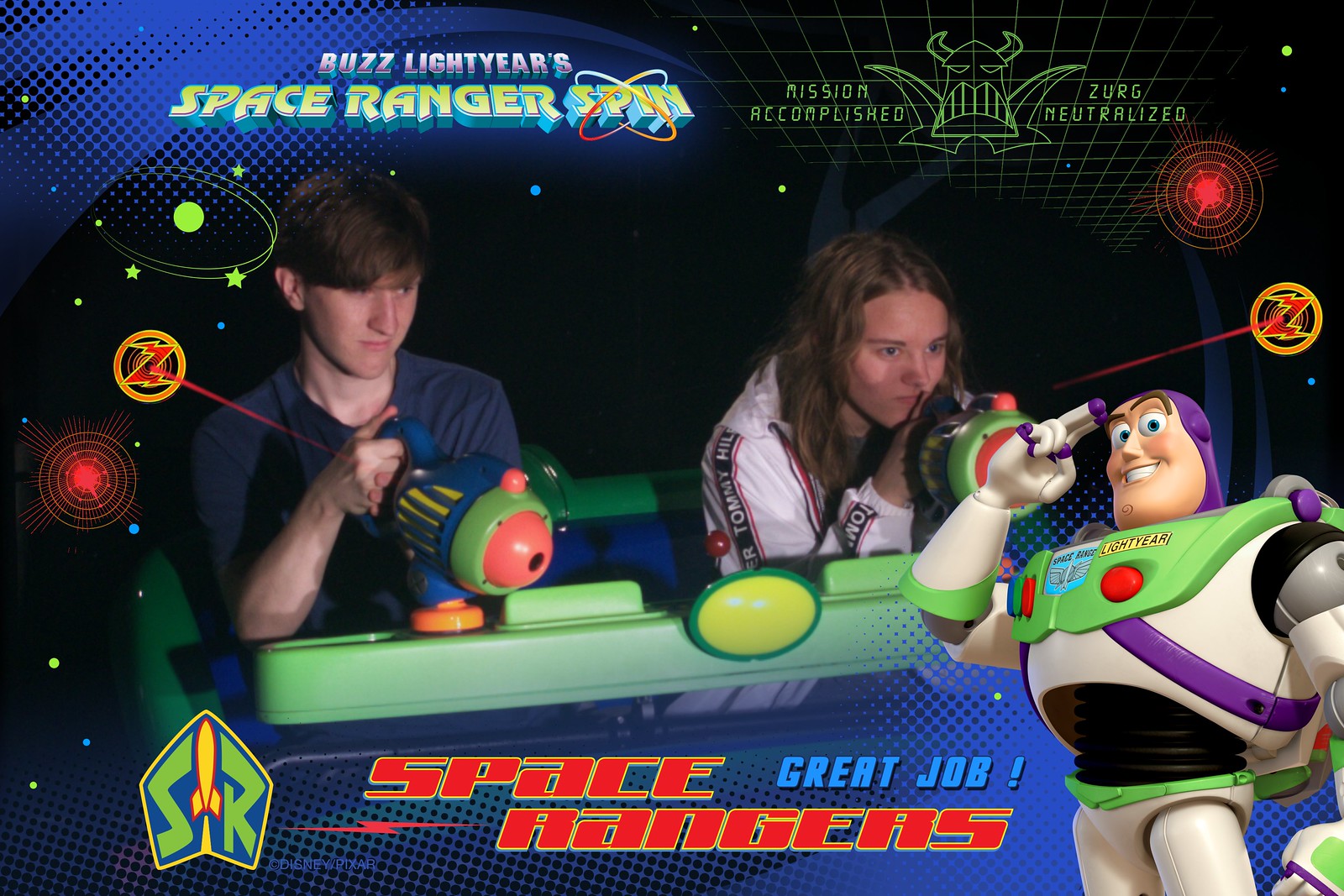In this vibrant and playful photograph, two teenagers, a young boy on the left and a young girl on the right, are deeply engrossed in a game. Both are wielding blue, green, and orange toy guns that resemble water guns, possibly part of a laser shooting game. The boy, a white male with brown hair, is dressed in a blue polo shirt, while the girl, a white female with long brown hair, is wearing a predominantly white jacket decorated with a black and white ribbon.

The setting is adorned with various colorful texts and graphics. Above the teens, the phrase "Buzz Lightyear's Space Ranger Spin" is prominently displayed, followed by "Mission Accomplished Zerg Neutralized," indicating a victorious end to their game by neutralizing the monster Zerg. Surrounding these words are stars, circles, and laser beam graphics, adding to the dynamic atmosphere. Notably, Buzz Lightyear himself makes an appearance in the lower right corner, saluting with two fingers to his eyebrows, standing confidently with a cartoon-like presence. Additionally, the bottom of the image confirms their success with the text, "Space Rangers Great Job."